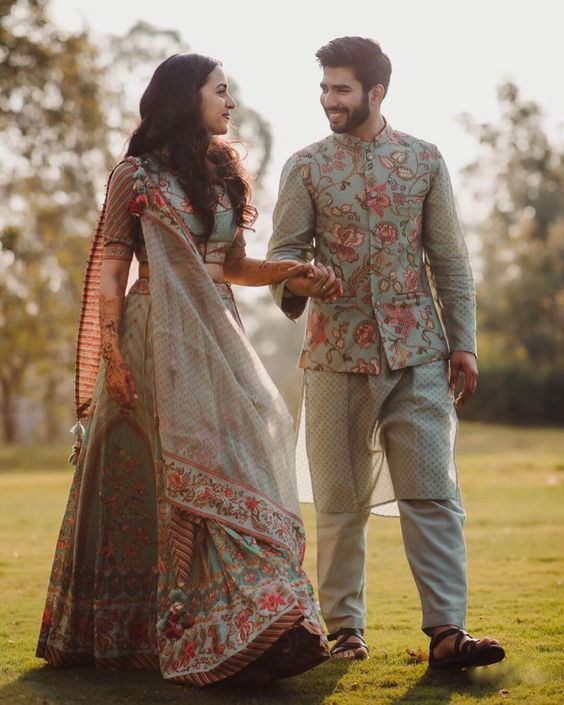The image showcases an outdoor setting with a blurred grey sky and trees in the background, featuring a couple holding hands as they walk through a grassy field. The woman, positioned on the left, has long, brown, wavy hair and is adorned in a colorful, heavily patterned traditional Indian wedding dress with reds and pinks and a drape over her shoulder that looks quite expensive. The man on the right, with short brown hair and a beard, is wearing a long-sleeve top with an olive-green hue and a floral pattern, paired with matching trousers and sandals. Both are smiling and gazing lovingly into each other's eyes, suggesting they are deeply in love. Their attire and the professional, staged nature of the photo strongly indicate that this is a wedding photograph, capturing a moment of joy and affection between the newlyweds.